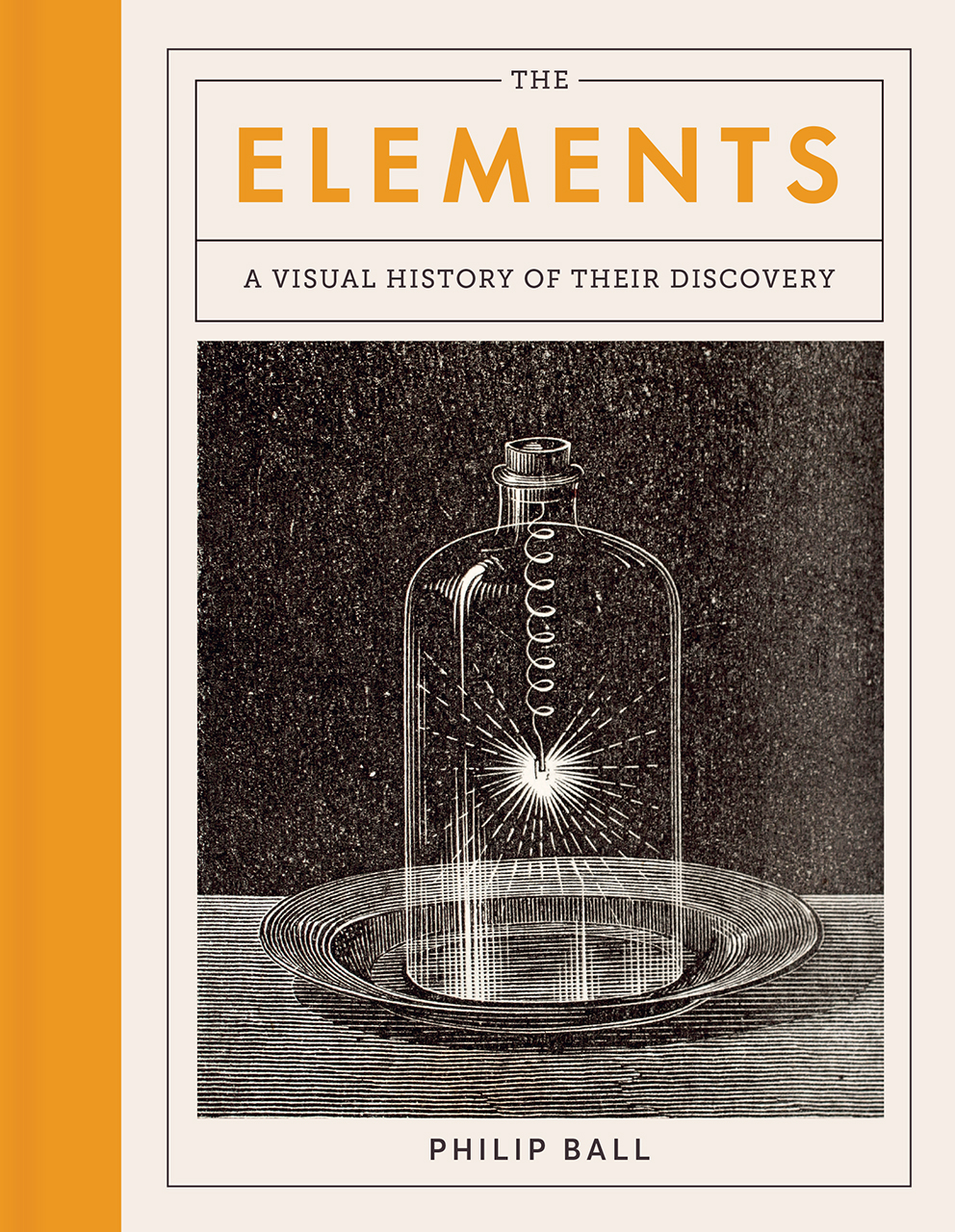The book cover of "The Elements: A Visual History of Their Discovery" by Philip Ball is a striking combination of black and white imagery with color accents. Dominating the cover is an intricate, sketch-like illustration of a primitive light bulb or energy experiment contained within a large jar, resembling a beaker. This jar is placed on a plate, which rests on a table, all set against a pure black background that emphasizes the delicate, almost pencil or charcoal-quality shading of the sketch. The title "Elements" stands out in a bold, large font in an orange hue, matching the orange trim running down the left edge of the cover. The meticulous details—including the radiating lights from the coil inside the bulb and the clean, visually appealing layout—give the viewer a sense of scientific discovery and historical depth.